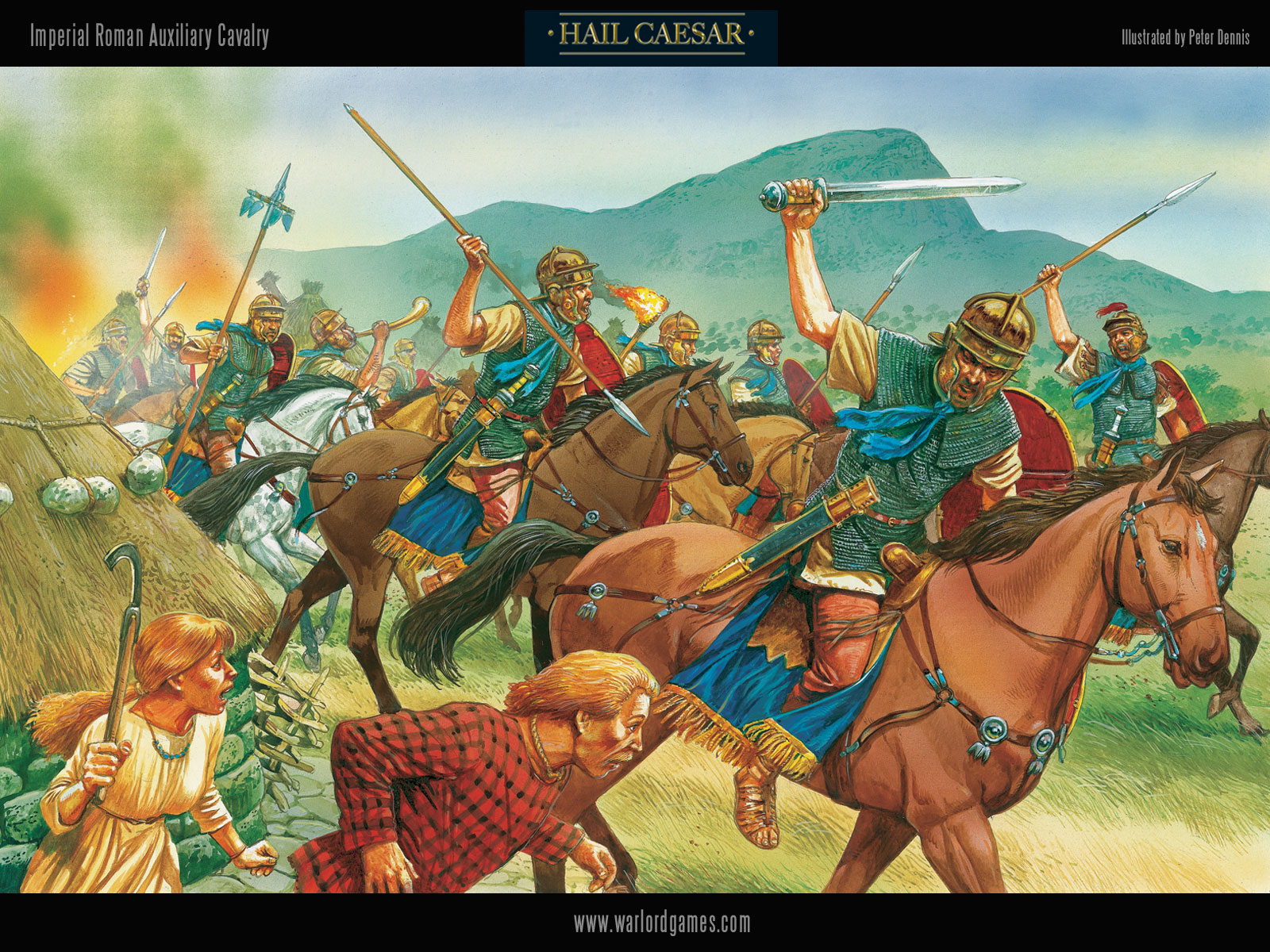The image is a detailed cartoon drawing of an action-packed scene depicting a cavalry charge. It is in a landscape orientation with solid black horizontal bands at both the top and bottom. In the bottom band, white text in the center reads "www.warlordgames.com." The top band features three distinct texts: "Hail Caesar" in raised gold text enclosed by horizontal lines and dots, "Imperial Roman Auxiliary Cavalry" in white in the top left, and "illustrated by Peter Deniz" in white in the top right.

The main illustration shows Imperial Roman Auxiliary Cavalry soldiers on horseback. The horses are mostly various shades of brown with one white horse visible. The soldiers are wearing yellowish tunics with dark green, sleeveless overlays, and gold-colored helmets that cover the sides of their faces. Blue scarves are tied around their necks. They are equipped with an array of weapons like swords, spears, multi-bladed weapons, and torches with flames. One soldier is particularly noticeable for blowing a long, skinny yellow horn.

The background is filled with greenish mountains, and the ground is covered in yellowish-green long grasses. Flames are visible on the left side, possibly indicating destruction caused by the soldiers. In the left foreground, two terrified villagers—a man and a woman—are seen fleeing. The man, with long blonde hair, wears a red and black plaid shirt and a necklace. The woman, with long blonde hair tied back, is dressed in an off-white dress and holds a farming scythe aloft. They run past a partially visible thatched hut with a grey stone base and a yellow straw roof, its conical shape cut off by the edge of the image. The villagers have expressions of horror, the woman’s mouth open as if screaming, adding a dramatic tension to the scene.